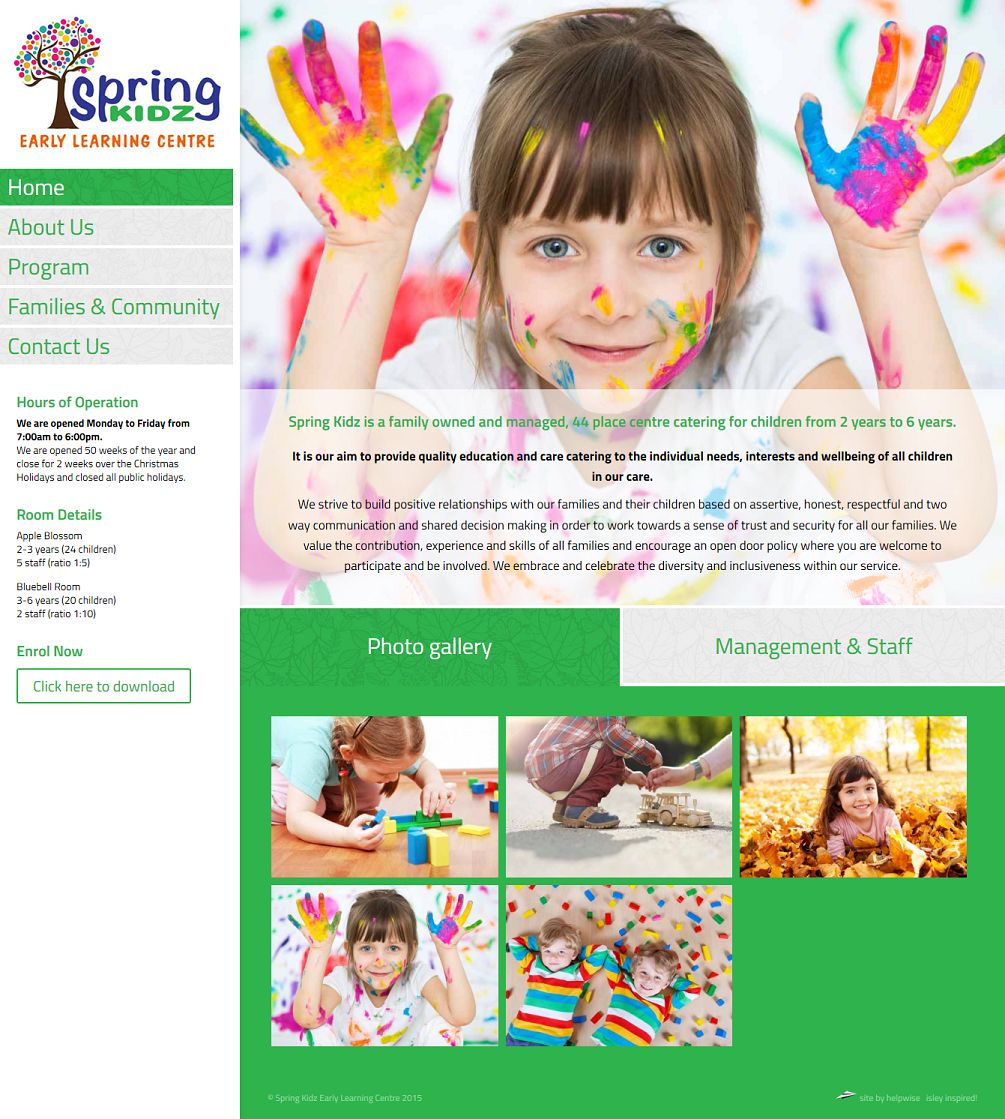In this vibrant image, a cheerful child with blue eyes is seen in the foreground, her face and nose adorned with colorful paints, mirroring the bright splashes on her hands. Her wide smile radiates excitement and joy. The backdrop text reads, "Spring Kids is a family-owned and managed center with a capacity for 44 children, catering to ages from two to six years. Our aim is to provide quality education and care tailored to the individual needs, interests, and well-being of every child in our care. We strive to build positive relationships with our families and their children based on assertive, honest, and respectful two-way communication and shared decision-making, fostering a sense of trust and security. We value our families' contributions, experiences, and skills, and maintain an open-door policy, encouraging active participation and involvement."